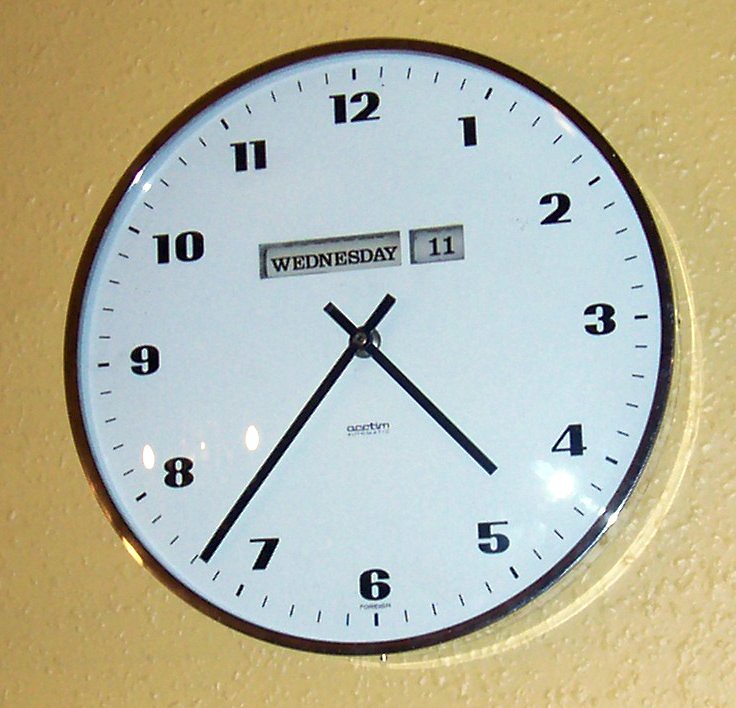In this detailed image, a circular wall clock with a black border is mounted on a yellow, bumpy-textured wall. The clock face features a white background with bold black numbers from 1 to 12, accompanied by small dashed lines marking 15-minute increments around the border. The clock prominently displays the day and date in two rectangular cutouts above the hands; the left cutout shows the day as "Wednesday," while the right cutout shows the date as the "11th," both set against a gray background. The black, rectangular hour hand points between the 4 and 5, and the minute hand points between the 7 and 8. Below the hands is the text "Actum." Additionally, there is a small reflection near the bottom right of the clock, emphasizing its glossy surface.